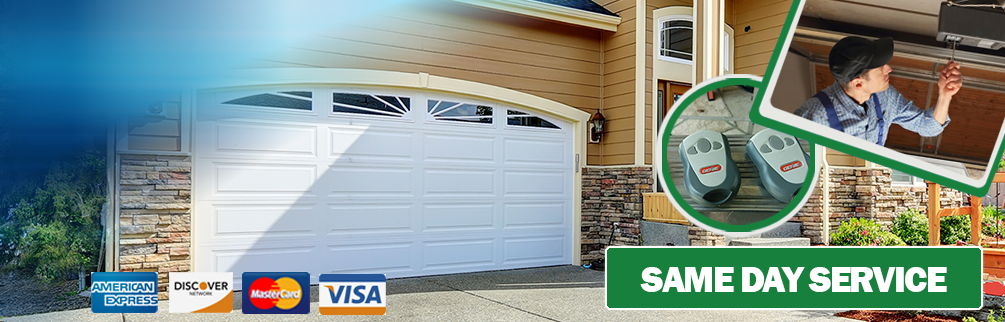The image displays a website that prominently advertises "Same Day Service" against the backdrop of a large house with a visible garage. The website indicates acceptance of American Express, Discover, MasterCard, and Visa for payments. The overall aesthetic features a blue and white color scheme, with a reflective, shaded overlay on the upper portion of the garage.

Further down the page, there are pop-ups obscuring part of the house, making it difficult to view the entirety of the structure. These pop-ups include the image of a man in a hat, overalls, and a button-down shirt, diligently working on a piece of equipment in a kitchen setting. Two circular icons also appear, believed to represent garage door openers.

In the background of the pop-ups, some shrubbery is visible along with a brick base of the house. Additionally, there appears to be a wagon or another type of outdoor tool, though it's partially obscured by the misplaced pop-ups. The company name is notably absent from the visible portions of the website.